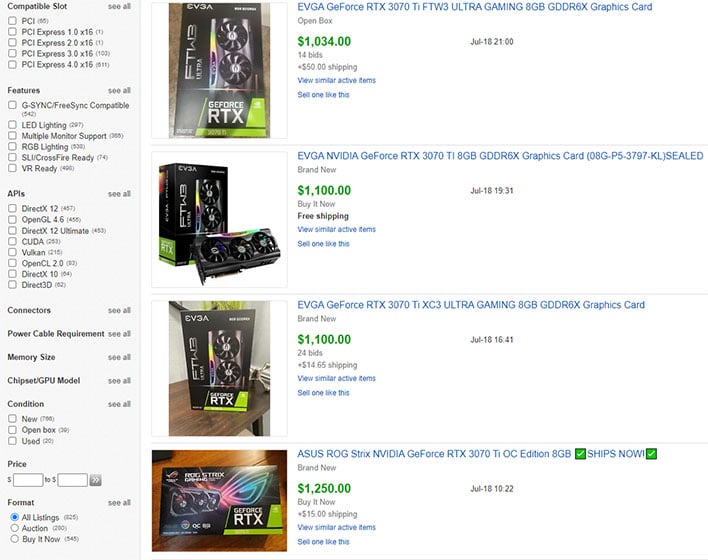Screenshot of a website selling computer hardware: 

At the top left, there is a navigation section offering a wide array of filter options:
- **Compatible Slot:** Options include PCI, PCI Express, PCI Express 2.0, PCI Express 3.0, PCI Express 4.0 x16 
- **Features:** Various features include G-Sync, FreeSync compatibility, LED lighting, multiple monitor support, RGB lighting, VR-ready capabilities, SLI and Crossfire readiness.
- **APIs Supported:** DirectX, OpenGL, DirectX 12 Ultimate, CUDA, Vulkan, OpenCL 2.0, DirectX 10, Direct3D.
- **Connectors, Power Cable Requirements, Memory Size, Chipset, GPU Model.**
- **Condition:** New, Open Box, or Used.
- **Price Range:** Customizable range from blank to blank.
- **Format:** Options for all listings, auction, or buy-it-now.

Displayed listings include variations of the EVGA GeForce RTX 3070 Ti FTW3 Ultra Gaming 8GB GDDR6X, offered at different price points.